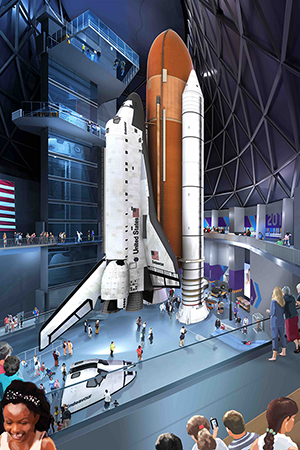This detailed artist's drawing depicts a white USA space shuttle, accented by a black tip and featuring visible United States flags on its side and wings. The shuttle is mounted beside a large orange cylindrical structure, which seems to represent the launching pad or a related support mechanism. This scene is set within a sizable gray indoor building characterized by a domed ceiling and multiple balcony levels, suggesting a possible museum or exhibition space. The blue floor is bustling with numerous visitors, with many individuals attentively observing and photographing the shuttle. Notable among the crowd is a black-skinned woman in the bottom left corner, wearing a white tank top and a distinctive black and white bow tie in her hair. Overall, the image effectively captures the sense of awe and attention drawn by this iconic space vehicle, thoughtfully detailed within an exhibition context.